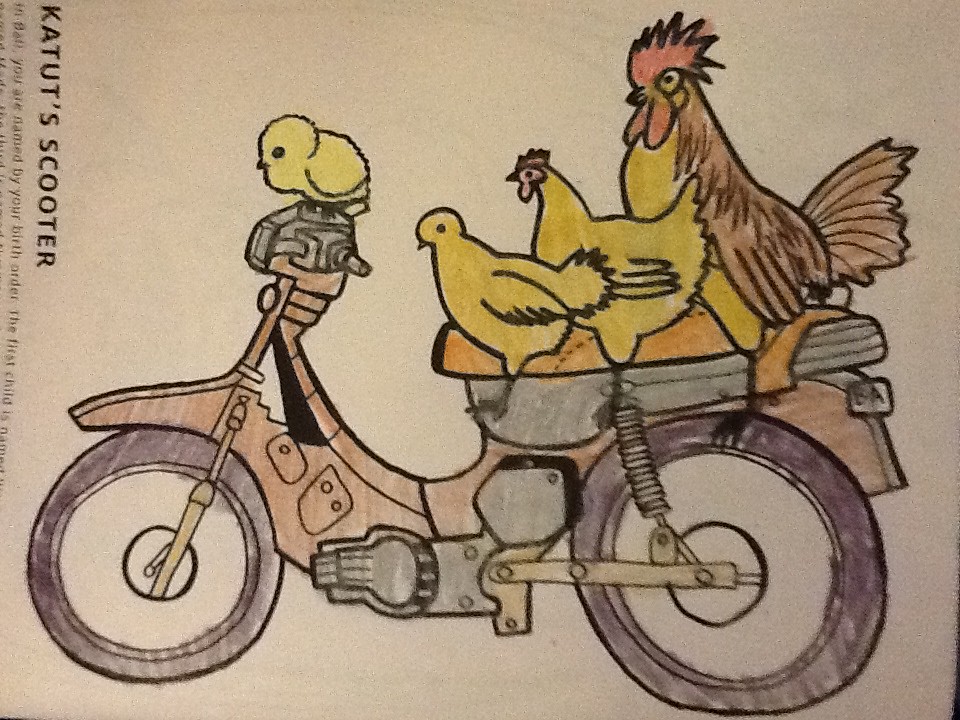The image appears to be from a children's coloring book, depicting a motorcycle, labeled "Katutz Scooter," ridden by a family of chickens. The motorcycle is drawn in black marker and colored primarily with colored pencils, showcasing a light brown body with dark purple or dark blue wheels and an orange seat. The chickens are positioned in birth order: a tiny yellow chick perched on the handlebars, two middle-sized yellow chicks on the front part of the seat, and a larger hen and rooster, identifiable by its brown feathers and distinctive red comb and wattle, sitting at the back. The rooster has a yellow belly, adding to its distinctive look. The background of the picture is left white, giving prominence to the detailed, mostly within-the-lines coloring done by presumably an older child. Additional faint text suggests something about naming by birth order, but it is incomplete and less legible. The drawing, oriented to the left, captures a lively and whimsical scene, perfect for a children's book.